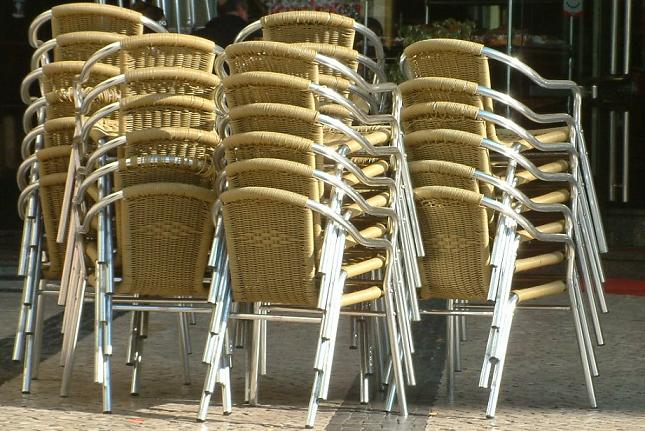This photograph captures a cluster of wicker chairs, neatly stacked in several tall columns. The chairs, each with an aluminum-tube frame and a woven wicker seat and backrest, exhibit a light tan to golden color, characteristic of rattan. Distinct horizontally-oriented diamond patterns embellish the backs of the chairs. Not all stacks are identical; some have six chairs, while others vary between five and eight, depending on the grouping. The stacks rest on a gray stone-tiled floor interspersed with broad, darker gray stripes or accents, potentially indicative of a decorative stone sidewalk or a restaurant patio. The background remains somewhat obscure, yet hints of a café environment can be discerned, with some glass doors and faint figures, including a person in a black hoodie, subtly visible. The photograph, taken in natural daylight, adds to the ambiance, casting soft shadows on the ground.